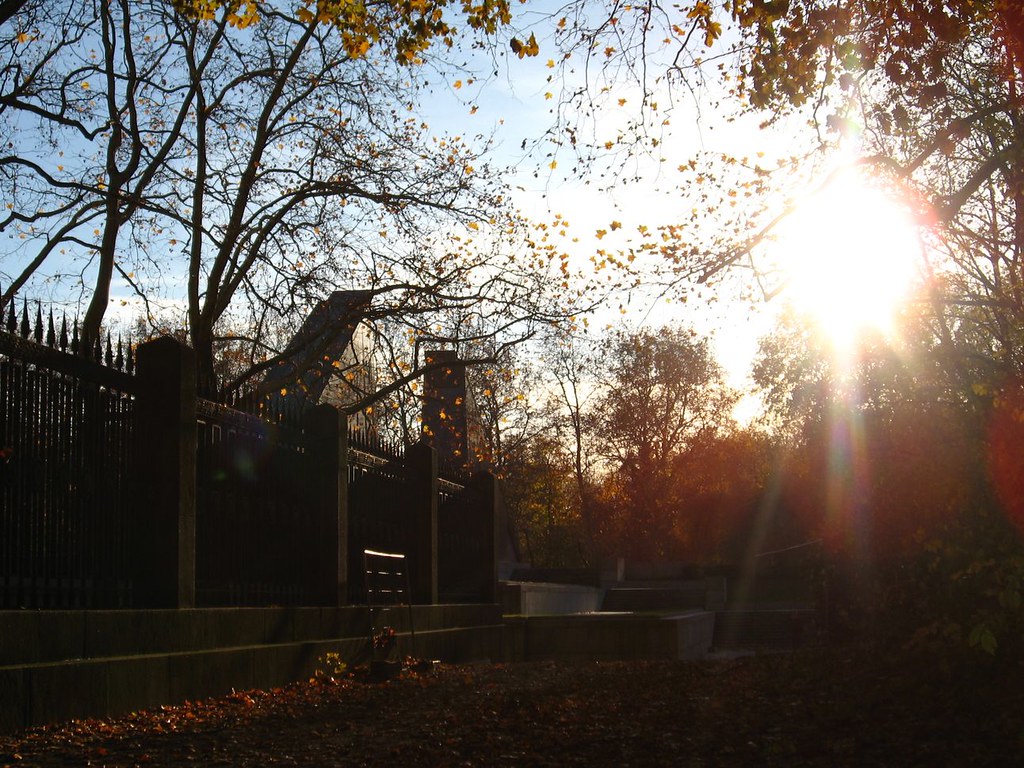The photograph captures the serene ambiance of an expansive park during the late afternoon in early fall. The sun, positioned low in the predominantly blue, lightly clouded sky, casts warm, blinding rays through the partially leafless branches of the trees, projecting dappled light and shadow on the leaf-strewn ground below. Dominating the left side of the image is a tall, wrought iron gate with pointed spikes, framed by cement pillars resting on a gray cement platform, extending into the distance. This structure gives the park a historical or classical feel, reminiscent of Central Park or potentially a cemetery, enhancing the scene's tranquil yet slightly somber atmosphere. Scattered across the ground are vibrant remnants of fall foliage in hues of orange, green, and yellow, alongside some flowers. In the background, subtle architectural elements, including a cement bench and distant buildings, hint at the park's vastness and its blend of natural and man-made beauty.